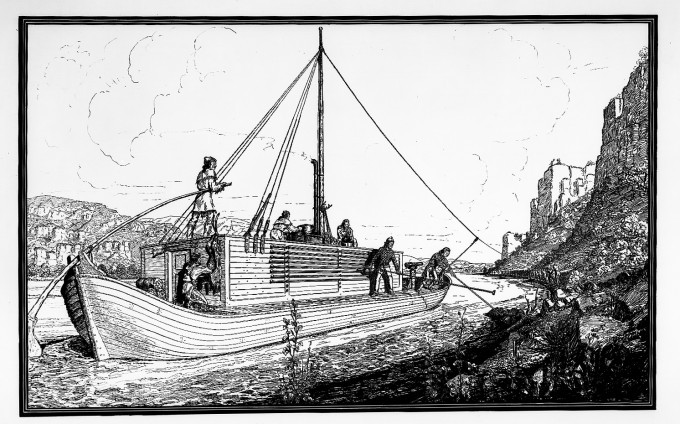This is a black and white pencil sketch, depicting a vintage wooden ship, likely from the 1700s or 1800s, navigating a narrow river towards a craggy island with adobe-type buildings. The ship features a central mast with wires extending to various parts of the boat. It may contain what appears to be a wheelhouse and possibly a steam engine, suggesting it could be a mid to late 1800s vessel, possibly a fireboat equipped with a nozzle and fire hose. Several men, potentially firemen, are seen on the boat, with some hanging off the sides and others on different deck levels. The shoreline is barren except for scattered rocks and a few plants; no people are visible in the distance. The sky is subtly shaded with makeshift clouds, adding depth to the entirely monochrome artwork of shadowed hillsides and serene landscape.